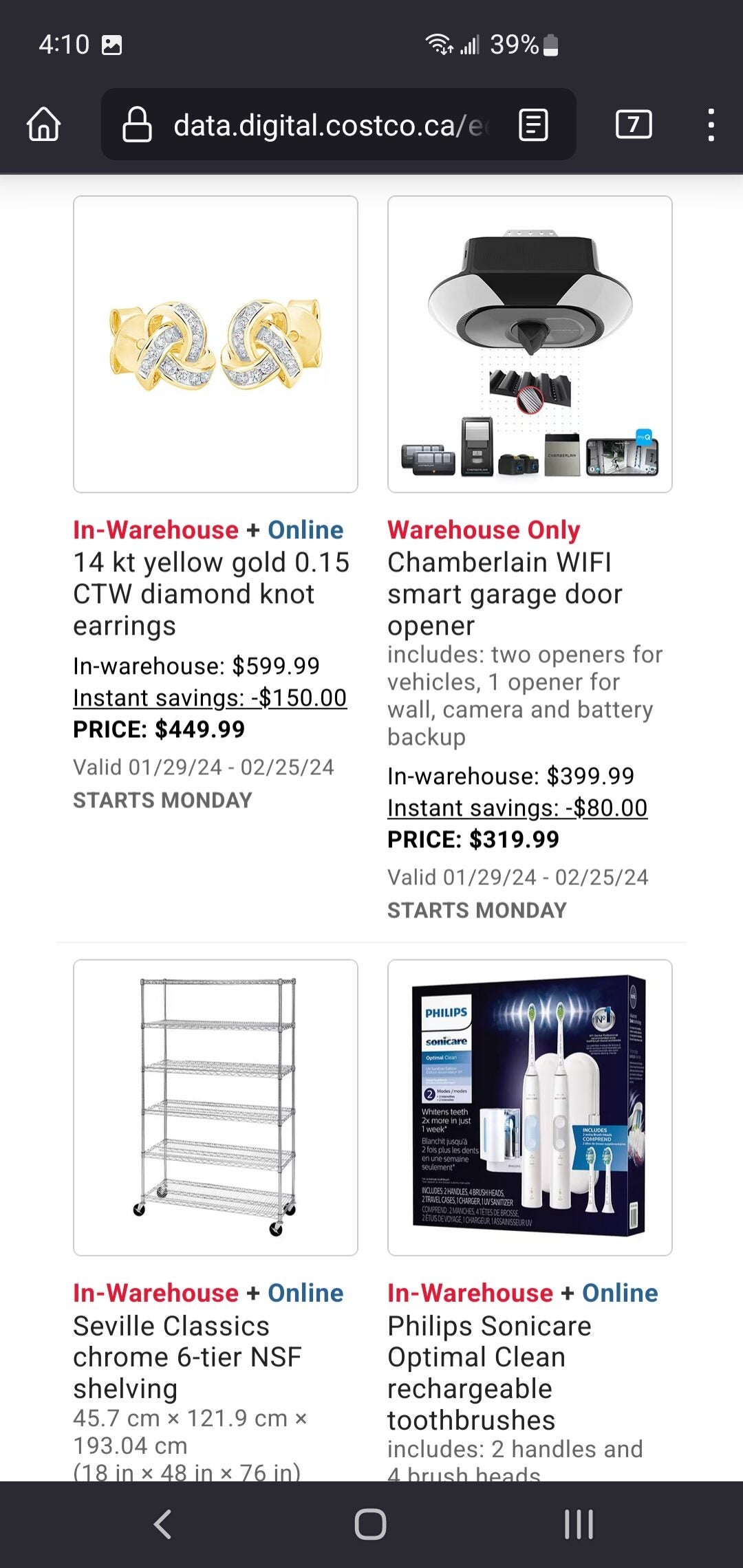A vertical rectangular image captured from a smartphone, with the top portion featuring a typical phone interface. The upper black border displays the time on the left, and icons for signal strength, Wi-Fi strength, battery percentage at 39%, and a small battery icon towards the center-right. Below this bar, a navigation bar with a home icon on the left, and the URL data.digital.Costco.ca along with additional icons on the right is visible, suggesting this is a screenshot of the Costco mobile app.

The main content below is divided into product listings, similar to a digital storefront. On the left, there are 14-karat yellow gold CTW diamond knot earrings with a listed price. On the right, a warehouse-only listing for a Chamberlain Wi-Fi smart garage door opener is displayed. Further down, a Seagull Classics chrome six-tier shelving unit is shown on the left, while on the bottom right, Philips Sonicare Optimal Clean Rechargeable Toothbrushes, which includes two handles and two brush heads, are featured. 

At the very bottom of the image, another black border displays three icons: a white left-pointing arrow, a square, and three vertical lines, indicating potential navigation or menu options within the app.